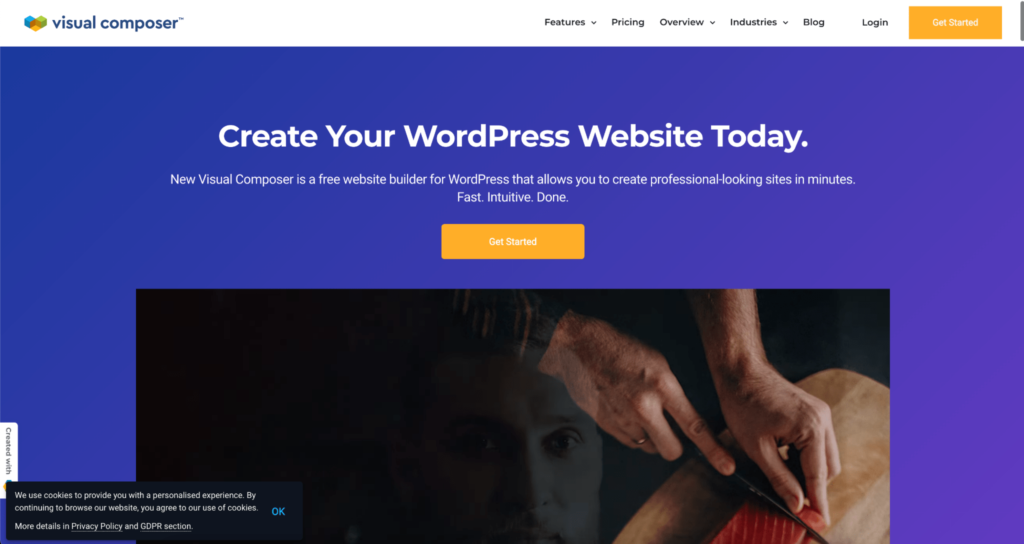The landing page appears to be for a service called Visual Composer, which is a free website builder for WordPress. The interface includes several navigational options on the right-hand side, such as "Get Started," "Login," "Blog," "Industries," "Overview," "Pricing," and "Features," each of which likely redirects to relevant sections of the site.

On the left-hand corner, the Visual Composer logo is prominently displayed above the tagline, "Create your WordPress website today." A brief description follows, stating that the new Visual Composer is a free website builder designed to help users create professional-looking sites quickly and intuitively. Below this description is an orange "Get Started" button, inviting users to begin.

An engaging image below the "Get Started" button features two hands cutting what appears to be a piece of salmon, or another type of fish, with someone possibly observing through a window or glass. This adds a visual element to the page, making it more inviting.

In the bottom left-hand corner, there is a notice about cookie usage, informing visitors that by continuing to browse the website, they agree to the site's use of cookies. A clickable "Okay" button in blue allows users to acknowledge and accept this message.